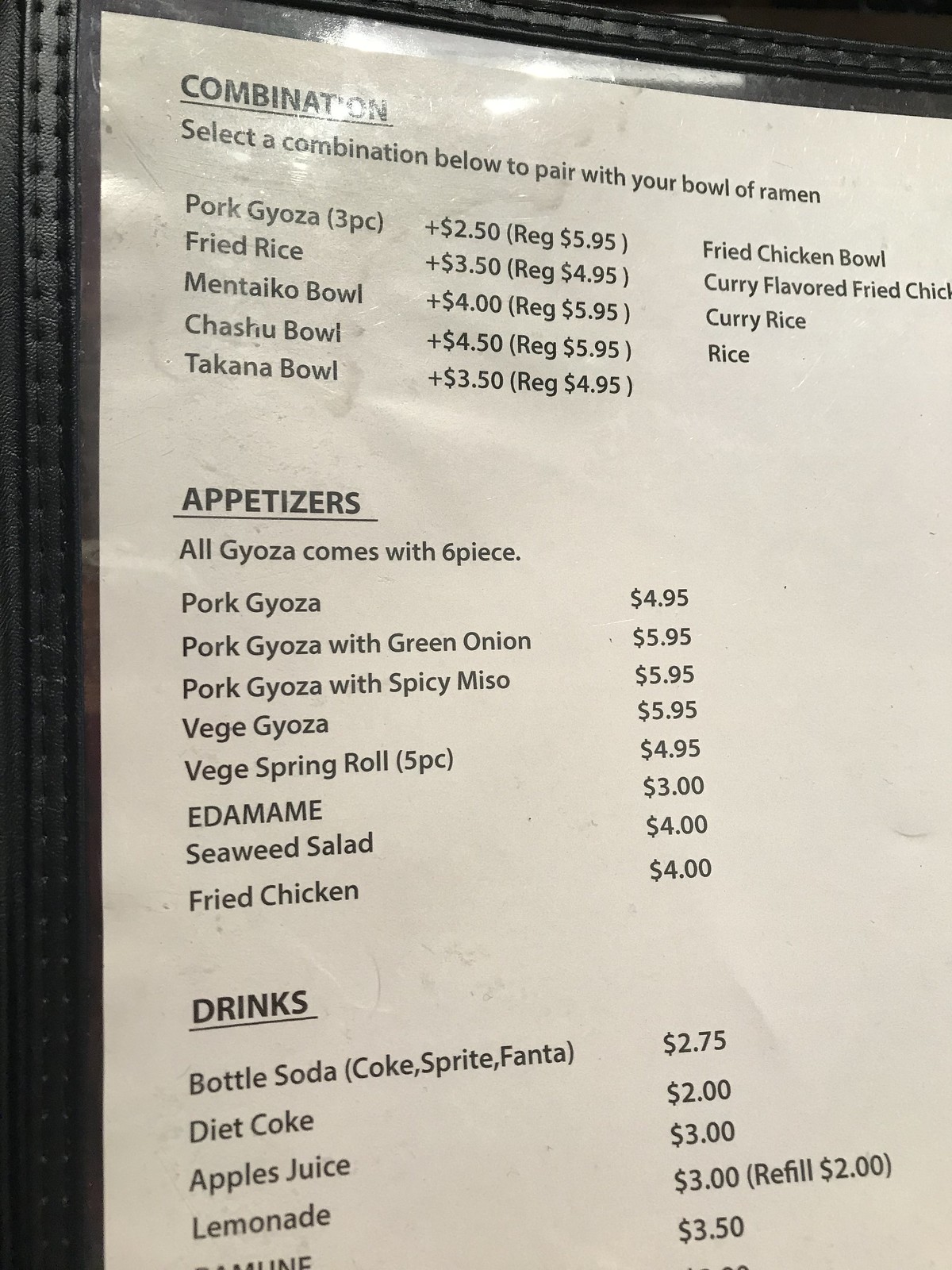A detailed photograph of a restaurant menu is presented, showcasing its offerings under the headers "Combination," "Appetizers," and "Drinks."

### **Combination**
Select a combination below to pair with your bowl of ramen:
- Pork Gyoza (Three pieces)
- Fried Rice
- Mentaiko Bowl
- Chashu Bowl
- Takana Bowl
- Fried Chicken Bowl
- Curry Flavored Fried Chicken
- Curry Rice
- Rice

### **Appetizers**
All gyoza orders come with six pieces:
- Pork Gyoza with Green Onion (Gyoza incorrectly spelled as "Gyozy")
- Pork Gyoza with Spicy Miso
- Vegetable Gyoza
- Vegetable Spring Roll (Five pieces)
- Edamame
- Seaweed Salad
- Fried Chicken

### **Drinks**
- Bottled Soda (Coke, Sprite, Fanta, Diet Coke)
- Apple Juice
- Lemonade

The visible range of prices on the menu shows that the most expensive item is priced at $5.95, while the least expensive item costs $2. Unfortunately, part of the menu is obscured and not visible in the photograph.